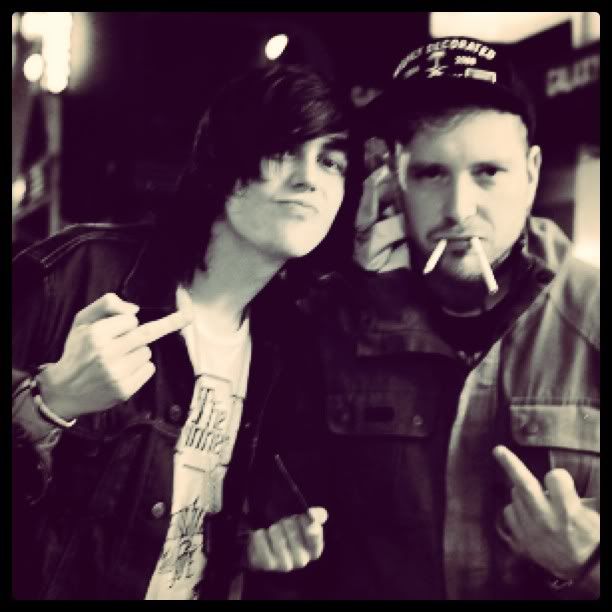In this black-and-white square photograph, bordered by a thick black edge, two young men are posed closely together, both flipping off the camera. The man on the left has long, dark hair partially covering his right eye and is dressed in a black leather jacket over a white t-shirt with an indistinct design. He is holding an unknown object in his left hand while giving the bird with his right. The man on the right, wearing a black baseball cap inscribed with the word "decorated" in white print, has two cigarettes hanging from his mouth and flips off the camera with his left hand. His attire consists of a tan jacket layered over a black t-shirt. Both individuals sport serious expressions. Centered over the image is a watermark reading "Photobucket" accompanied by a circular logo, followed by the phrase "Protect more of your memories for less" in a gray rectangle.